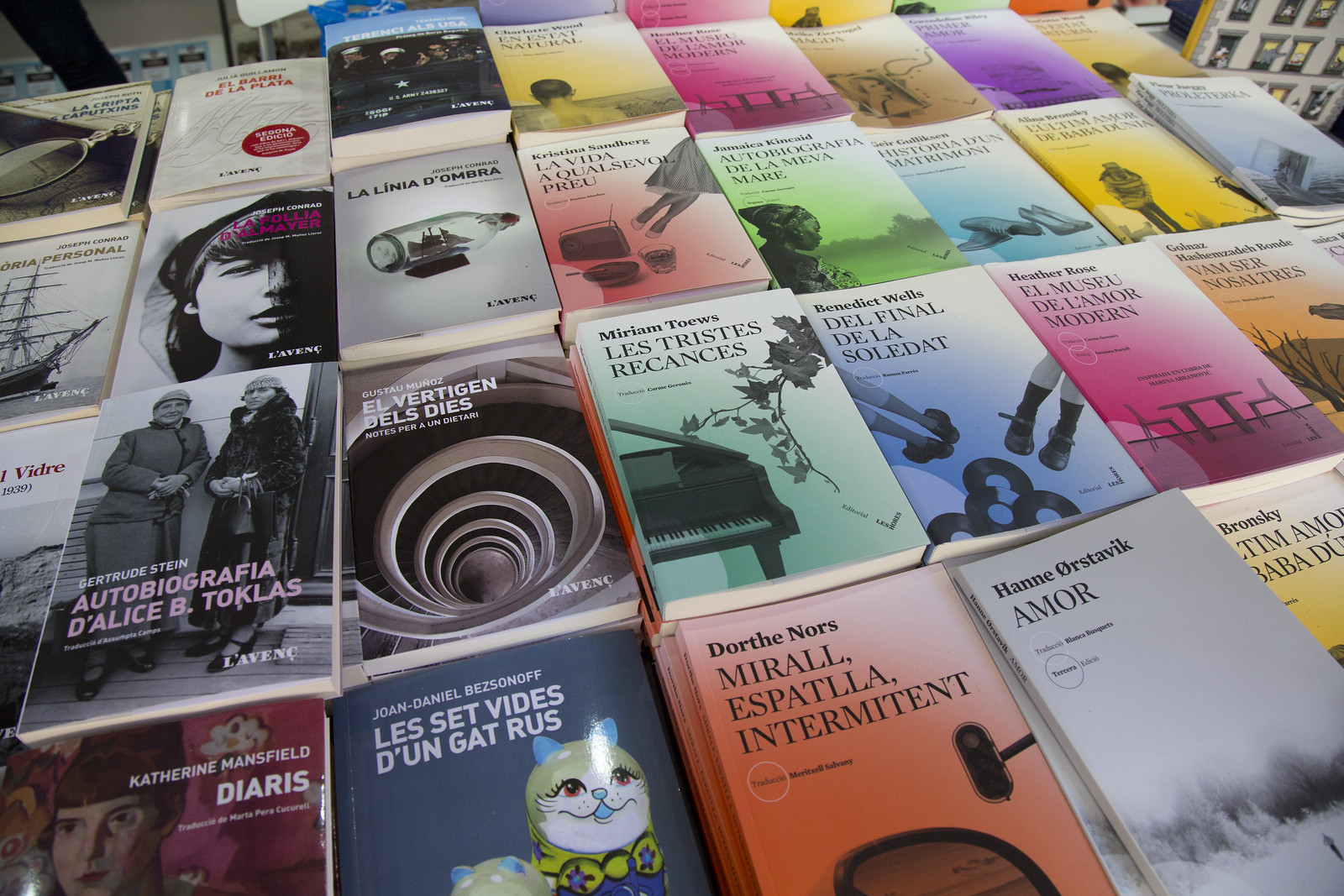The image depicts a display table in a bookstore, meticulously covered with a diverse array of books. Dominantly, these books are paperbacks, though there might be a few hardcovers interspersed. Every book proudly displays its title in French, covering a variety of subjects. On the right-hand side of the table, a collection of books stands out with a similar design: each features a gradient colored background—ranging from blue, red, yellow, to green—that transitions to white at the top. These books, likely part of a series, have their titles and authors marked in the upper left corner, paired with relevant imagery tinted by the gradient. In contrast, the left side of the table showcases a more eclectic assortment of individual titles and designs, each unique in its cover art. Among the recognizable titles are "La Polla Palmera," "La Nina de Ombra," "La Vida a Cua Se Vol Perdu," "Autografia de la Mera," and "Historia de Matrimonio." The overall scene is a colorful testament to the breadth of French literature available in the store.